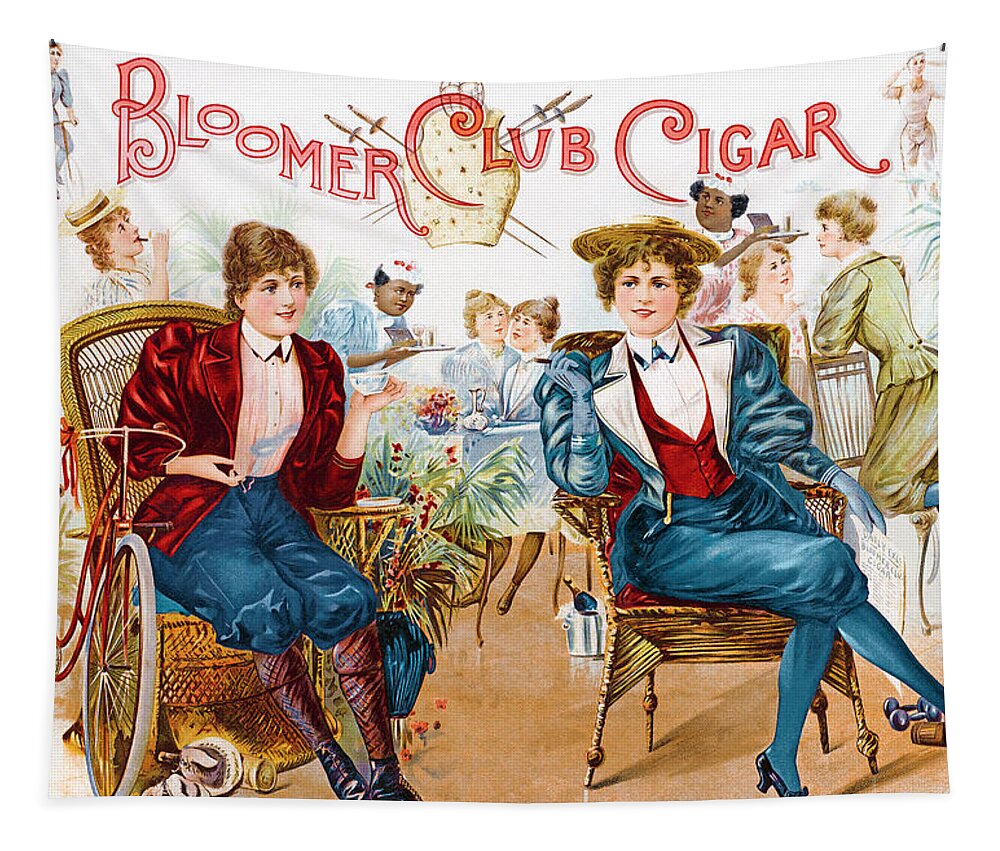This animated poster or banner features an advertisement for "Bloomer Club Cigar" written in red at the top. The setting appears to be from the 1920s, with white walls and a tan floor. Prominently, two women are seated in wicker chairs in the foreground. 

The woman on the left wears a red coat over a white undershirt, coupled with blue pants, dark socks, and black shoes. She is holding a white cup of tea and sits next to a red bicycle with white wheels. On the right, another woman is dressed in a blue coat, a red vest, and a white shirt with a blue bow tie. She is also wearing blue pants and blue socks with black shoes. This woman holds a cigar in her right hand. Both women share a similar appearance, down to their seated posture in brown wicker chairs.

In the background, a few more women are visible. Two black women, dressed in blue and pink with white headpieces adorned with red, are serving drinks and cigars. Amongst them, there are also white women seated and conversing. One white woman on the far left, wearing a white hat with a gold ribbon, is smoking. The background is further detailed with a black vase holding red flowers and green leaves, and a silver tin containing a champagne bottle with a gold top.

Under the main title, there is a shield with four swords crossing through it, featuring brown handles and gold or silver blades, adding a touch of ornamentation to the historical scene.